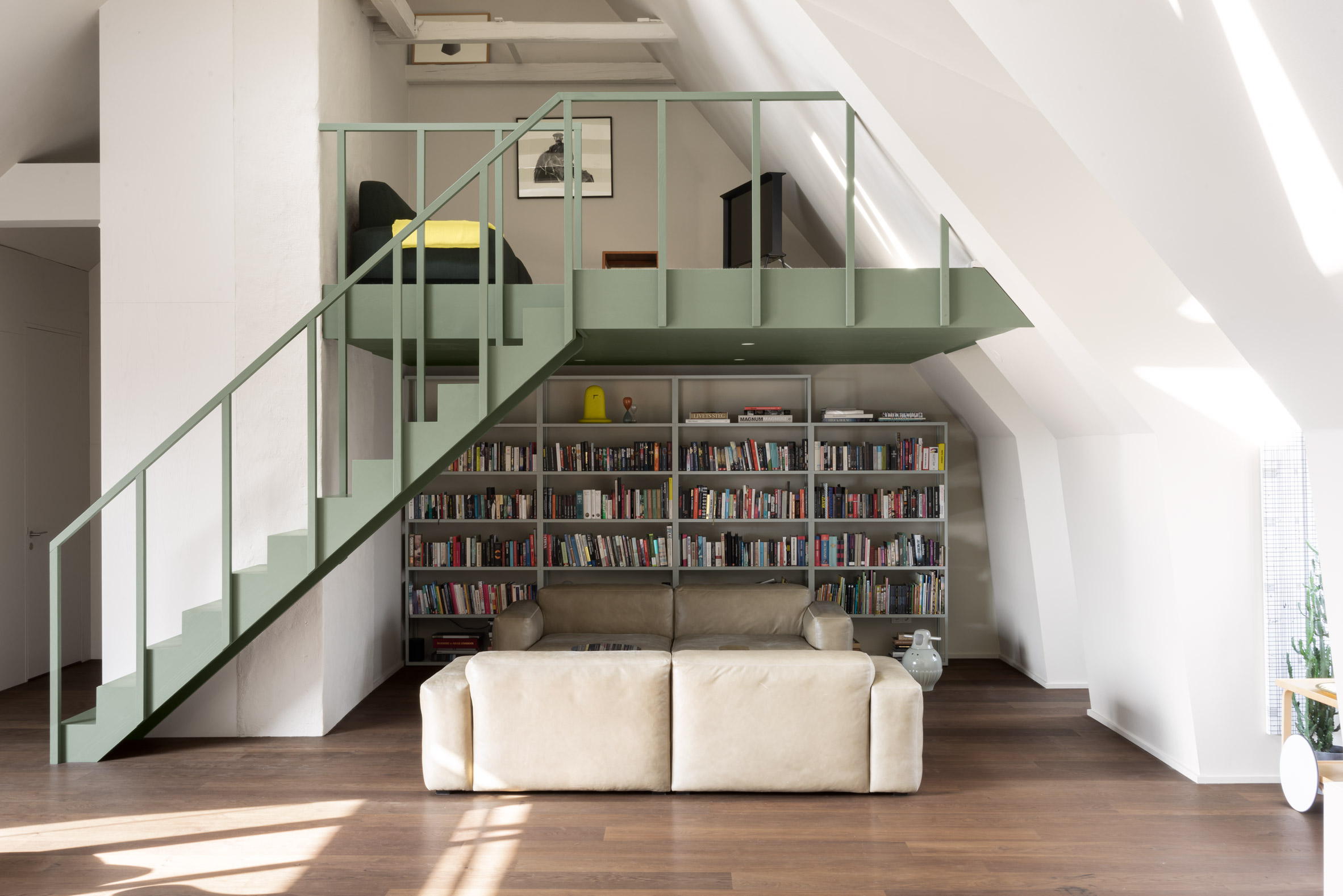This photograph captures a modern, architecturally distinctive living space with a horizontal-rectangular orientation. The room features walls that slant upward, creating a loft area with a triangular design, reminiscent of an attic. Central to the image is a green-painted wooden staircase that ascends to a loft platform. Below the loft, a large white bookshelf, fully stocked with various colored books, spans the entire width of the wall. The loft area itself is furnished with a black couch facing a flat-screen TV and is adorned with a picture in a brown frame. The living space boasts tall, vaulted, white walls and a wooden floor, possibly laminate. On the ground level, two tan-colored double-seated couches face each other, with one couch positioned with its back towards the bookshelf and the other facing into the nook. Light filters through a window on the left, illuminating a small alcove area with an upper shelf, though its contents are obscured. The overall design emphasizes an inviting, multifaceted area ideal for reading, relaxing, and entertainment.